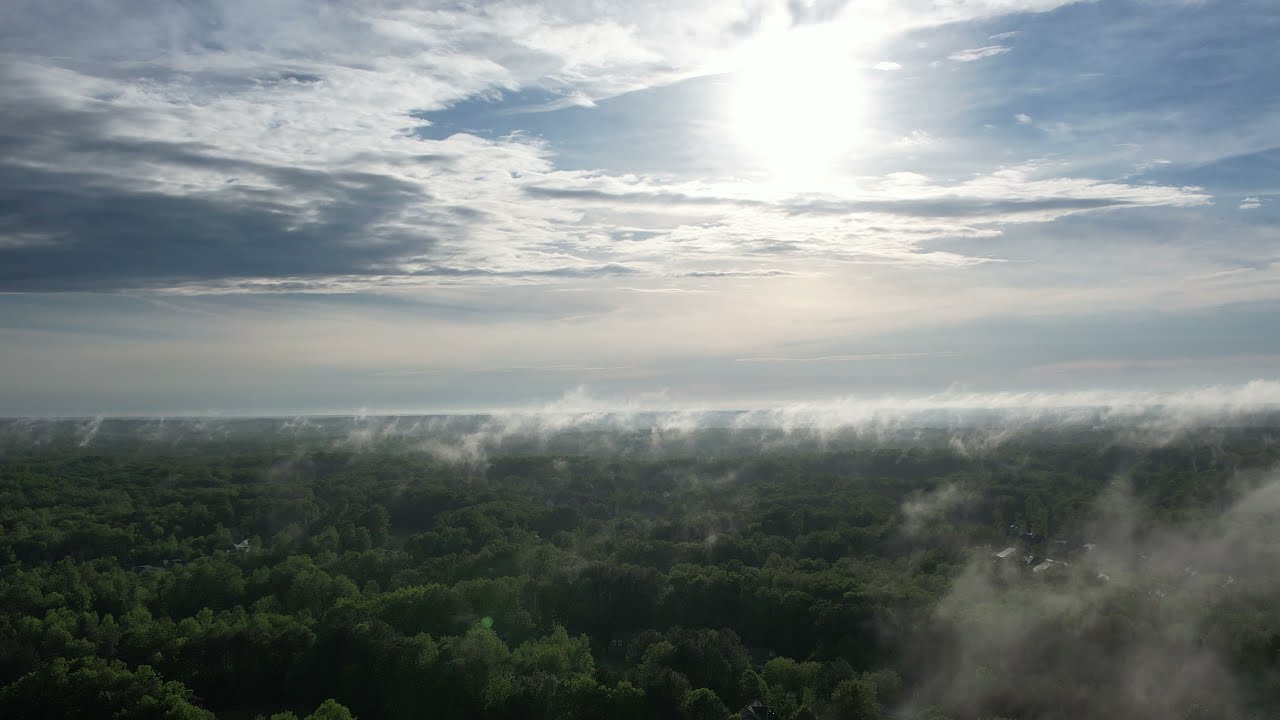The image captures a stunning, expansive outdoor scene viewed from a high vantage point. Dominated by a clear blue sky, a bright yellow sun shines prominently in the upper part of the image. A large cloud formation, stratus-shaped, is situated in the upper left corner, casting a slight haze toward the horizon. Greenery, mainly tops of trees from a dense forest canopy, stretches beneath the sky. There is a light mist hovering above the trees. Off to the right mid-area, silvery or grayish rooftops suggest the presence of homes, while a white-colored building is faintly visible center-left. In the lower part of the image, there is a captivating water feature that appears to be a waterfall cascading down a cliff, with foaming water flowing into a bluish-gray basin. The horizon shows minimal topographical change, hinting at the possibility of an ocean or sea in the distance, giving the scene depth and an open, airy feel.